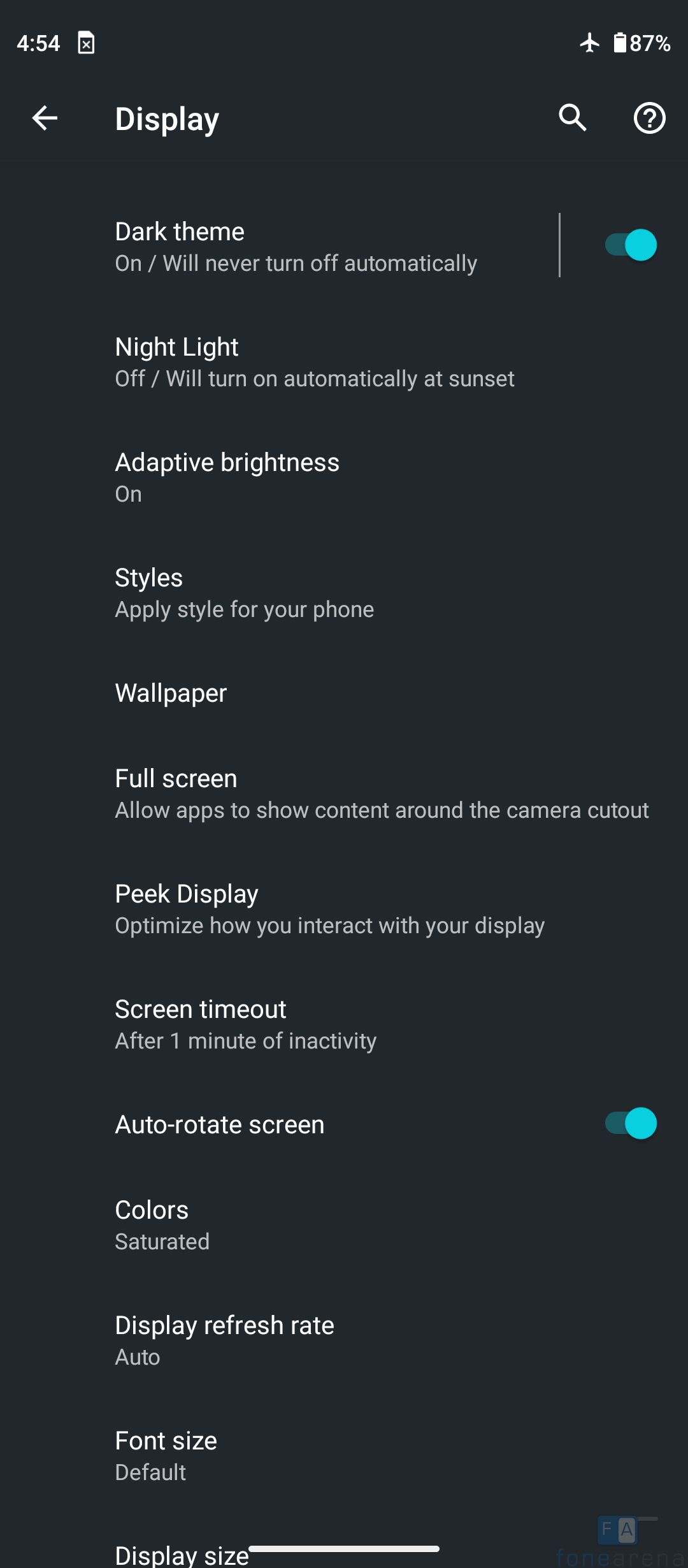This screenshot captures the "Display" settings menu from a smartphone. The background of the screen is black. Centrally positioned at the very bottom, slightly extending below the visible area by about a quarter of an inch, there is a small white horizontal bar. In the top-left corner, the time is displayed as "4:54" in white text next to a white-outlined square with a black interior. On the right side of the top bar, from right to left, it reads "87%", followed by a battery icon, and then an airplane mode icon pointing upwards.

Beneath the time, in the top-left, there is a left-pointing white arrow. To its right, the word "Display" appears in bold white text. On the right-hand side, there is a black circle with a white border and a white question mark inside it, and to the left of this circle is a search icon.

Underneath the "Display" heading, larger white text reads "Dark theme," with smaller gray text below it stating "On / Will never turn off automatically", followed by a vertical line and a teal toggle switch indicating it is active. The next items listed are "Night Light" with a line underneath, and "Adaptive brightness."

Further down, various settings categories are listed, including "Styles for your phone," "Wallpaper," "Fullscreen," "Peek display" (each with lines underneath), and "Screen timeout" which specifies "After one minute of inactivity." The "Auto-rotate screen" option indicates it is toggled on, and the list continues with "Colors" set to "Saturated," "Display refresh rate" set to "Auto," "Font size" set to "Default," and "Display size." The content spills off the bottom edge of the screenshot, cutting off some information.